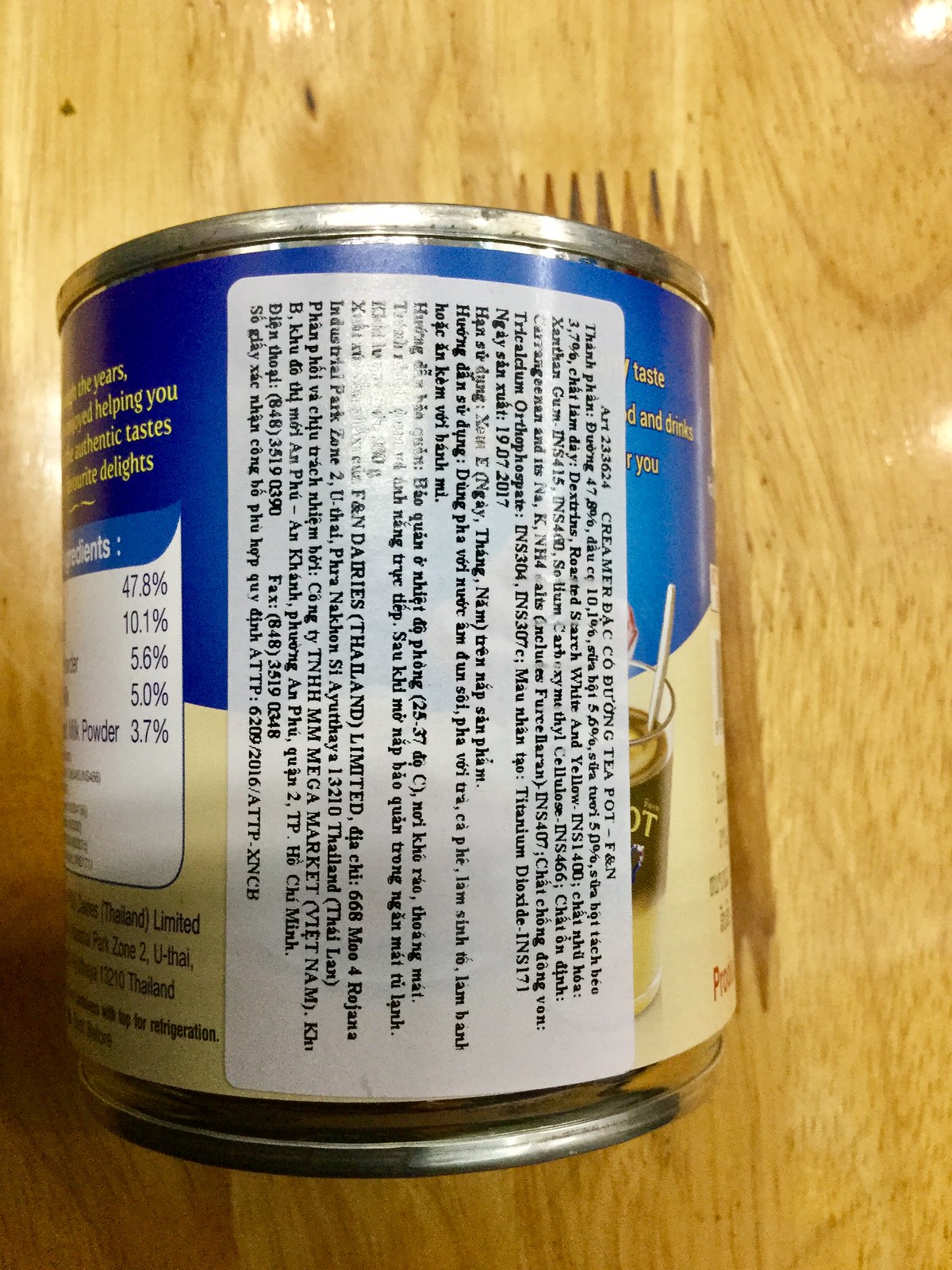The image depicts a cylindrical can lying flat on its side atop a light-colored, tan wooden counter. The can features a silver top and bottom, and it has a blue label at the top with a light yellowish color at the bottom. On the right side of the label, the word "ingredients" is prominently visible in blue text, followed by percentages in white text such as 47.8, 10.1, 5.6, 5.0, and 3.7, likely indicating daily value percentages. Behind the can, there appears to be a drink with brown liquid, a coffee mug, and a white straw hanging out of the drink. The can's backside shows a black text on a white rectangular label, but the text is too small to read. The detailed placement and additional elements suggest this might be a product like coffee creamer, sweetener, or evaporated milk, intended for use as a milk substitute.